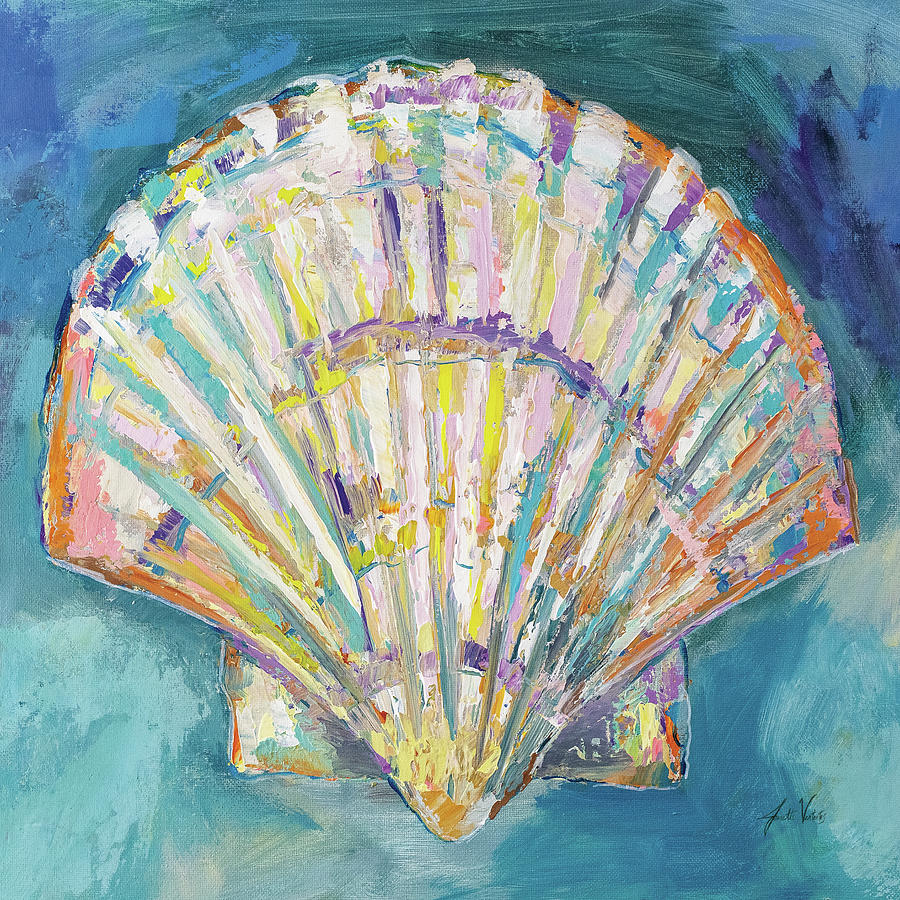The painting depicts a beautifully detailed, multicolored seashell against a blue and turquoise background. The shell, centrally positioned, boasts an array of colors including white, light blue, turquoise, yellow, orange, red, and purple. It is a perfect specimen with distinctive ridges along its surface, tapering down to a rounded point that creates a V shape at the bottom. The background features varying shades of blue, with visible brush strokes adding texture and depth, suggesting the subtle motion of water. The artwork, likely created with oil or acrylic paints, is signed by the artist in the bottom right corner, written in black.